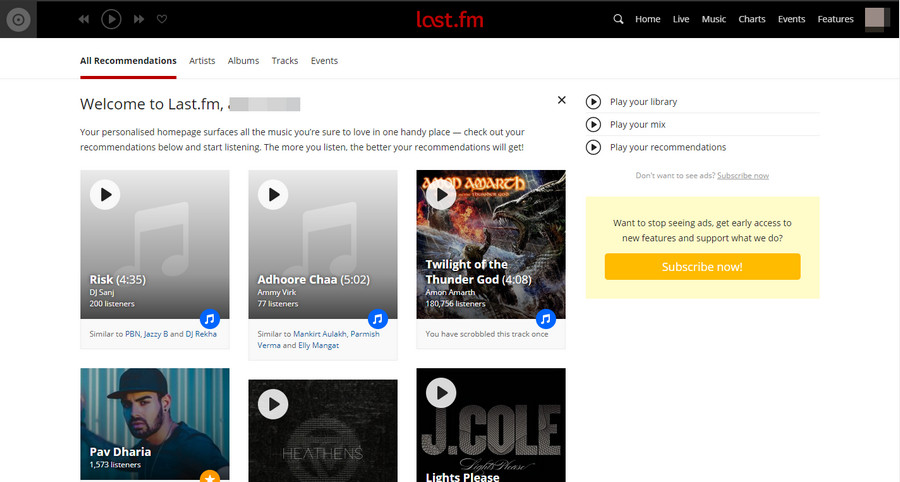The screenshot from the Last.fm music website, displayed on a widescreen desktop interface, prominently features a control bar at the top-left corner, complete with a play button flanked by back and forward buttons. At the top-right corner, there are several navigation links, including Home, Live, Music, Charts, Events, and Features, along with a search icon.

The webpage is currently open to the "All Recommendations" tab, part of a series of tabs that include Artist, Albums, Tracks, and Events. This tab contains a personalized welcome message from Last.fm, inviting users to discover music tailored to their tastes. The message reads: "Welcome to Last.fm. Your personalized homepage surfaces all the music you are sure to love in one handy place. Check out your recommendations below and start listening. The more you listen, the better your recommendations will get."

Below this welcome note, the page showcases six distinct music recommendations, spanning various artists, albums, or tracks. These recommendations appear to be diverse, suggesting a range of musical genres or styles, underscoring Last.fm's effort to cater to the unique preferences of each user.